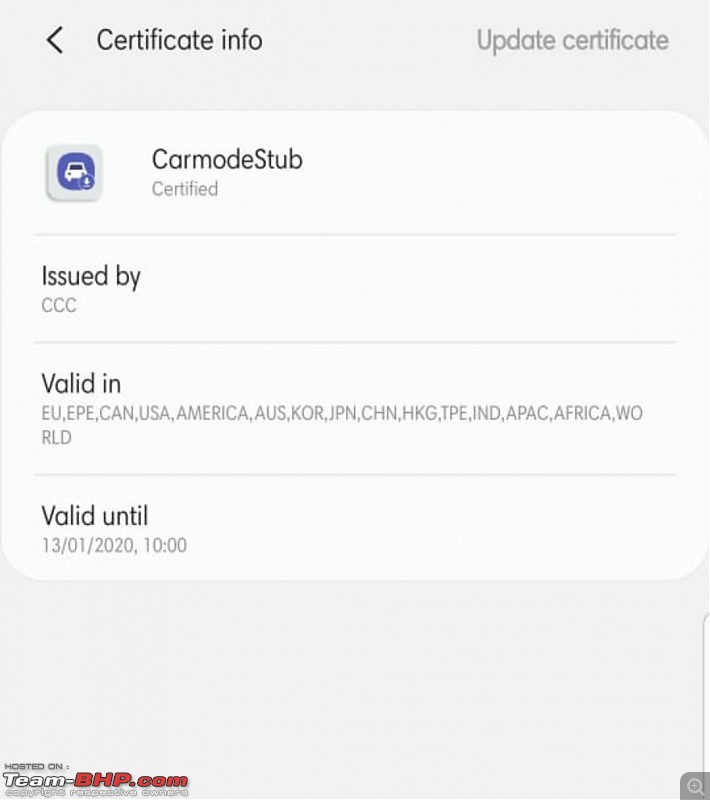A clean, orderly screenshot showcases certificate information within a mobile app. The backdrop is a subtle light gray. At the screen's top, the title "Certificate Info" appears in prominent black text with a left-pointing arrow, while the top right corner displays "Update Certificate" in dark gray lettering. 

Central to the interface is a white, rounded-corner rectangle divided into four horizontal sections. The uppermost section houses a smaller gray rectangle with softened edges, overlaid by a blue, rounded-corner rectangle depicting a white, cartoonish icon of a car front-view. Adjacent to this icon, "Car Mode Stub" is written, followed by "Certified" in light gray text.

The second section reads "Issued by CCC." The third section lists an extensive range of regions where the certification is valid: EU, EPE, CAN, USA, America, AUS, KOR, JPN, CHN, HKG, TPE, IND, APAC, Africa, and World. The final section notes the validity period, "Valid until 13/01/2020, 10:00."

At the screen's bottom left, a logo in white text asserts "Hosted on team-bhp.com," with "team-" written in white and "bhp.com" in red, accompanied by "Copyright Respective Owners" beneath it. On the bottom right, a gray rectangle with a single rounded corner holds a magnifying glass icon featuring a plus sign.